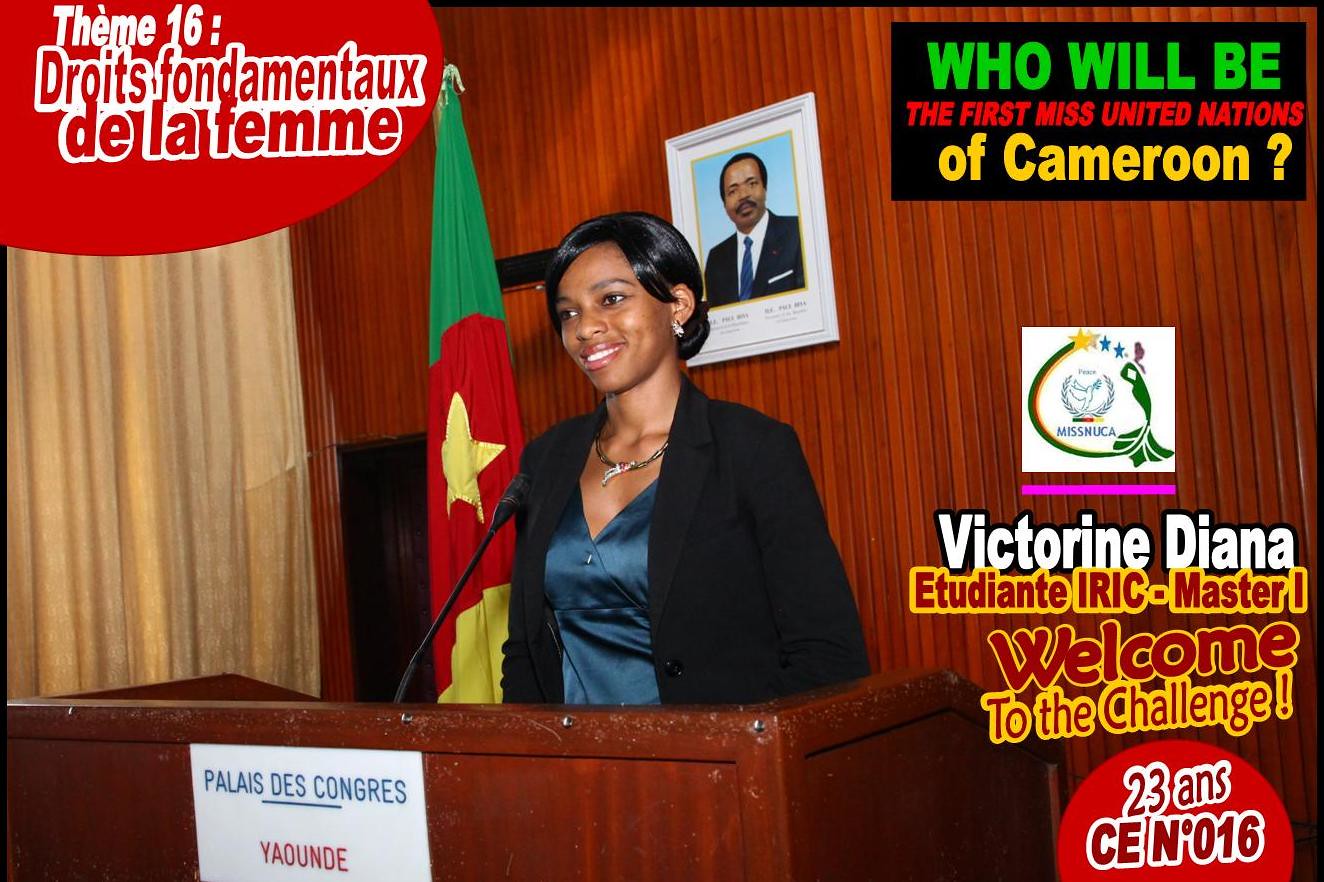In this image, a smiling African-American woman with short, shiny dark hair stands behind a redwood podium, dressed in a black blazer over a blue dress, accentuated with a necklace. She has dimples and dark eyes, and she is gesturing towards the left. The podium features a white sign reading "PALAIS DES CONGRES" with "YAOUNDE" in red letters beneath it. Behind her is a backdrop of redwood paneling, and to her left is a green, red, and yellow flag with a yellow star. An image of an African-American man with a mustache wearing a suit hangs on the wall behind her. The setting is further detailed with the text "Who will be the first Miss United Nations of Cameroon?" prominently displayed along with "Victorine Diana, Utante IRIC Master 1, Welcome to the challenge." A microphone stands before her as she addresses the audience.